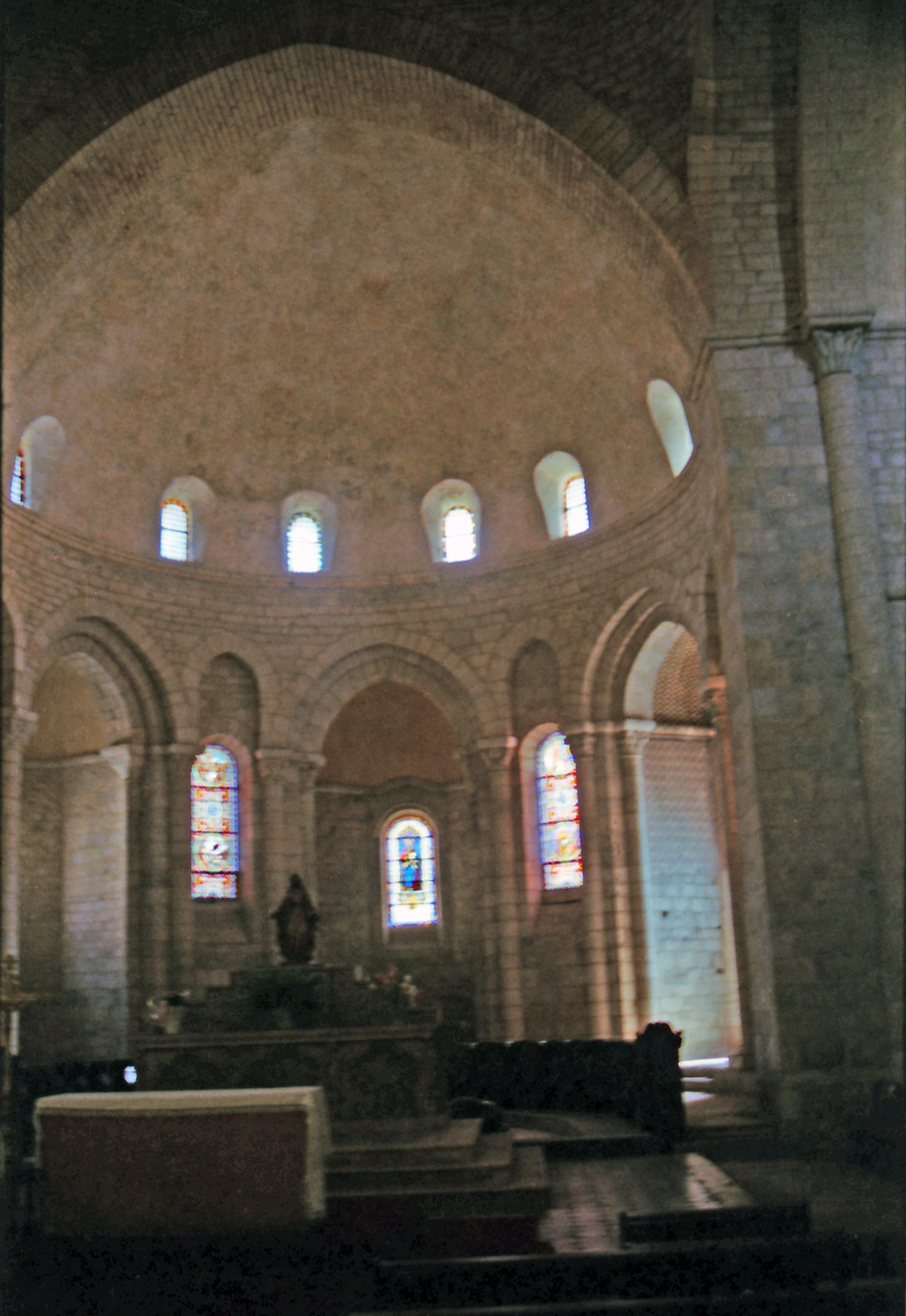This image captures the sanctuary of an old church, likely a basilica or cathedral, featuring a richly detailed architectural setting. The large, dome-shaped ceiling, constructed from creamy-colored stone, is adorned with stained glass windows that circle the top, allowing multi-colored light to filter through and illuminate the interior. Below the dome, a series of grand pillars and arches frame the space, with additional stained glass windows fitted within the arches. The walls are predominantly made of brown stone or brick, contributing to the historical ambiance of the structure. The altar, located at the back, is accessible via a set of dark steps and is characterized by a railing and a statue that could represent either the Sacred Heart of Jesus or the Immaculate Heart of Mary, though it's hard to determine due to the low light conditions. To the right side of the nave, there may be a baptismal font, while light streams in from what could be a large window or an open door. Altogether, this sacred space, complete with a cuboidal-shaped tomb and intricate designs, exudes a serene yet solemn atmosphere, accentuated by the blend of natural and stained glass lighting.